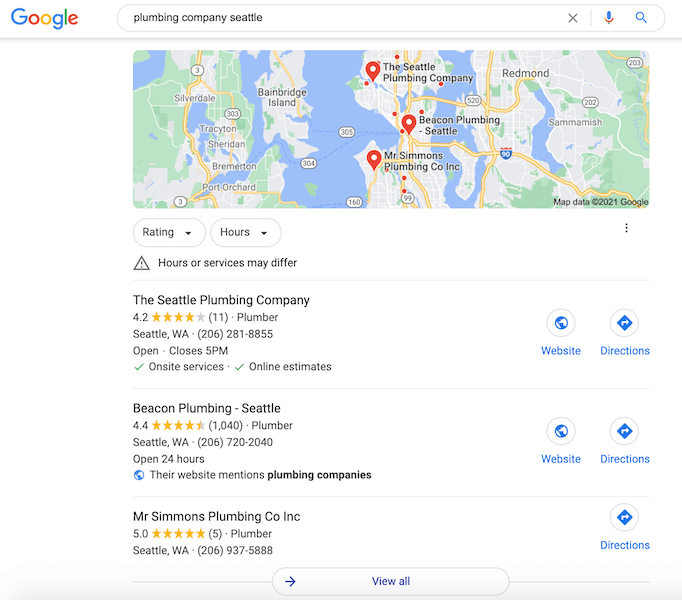The image displays a Google search results page for "Plumbing Company Seattle." Prominently featured at the top is the iconic Google logo in red, blue, green, and yellow, followed by a search bar with the query "Plumbing Company Seattle." Adjacent to the search bar are a gray "X," a multicolored microphone icon in gold, red, and blue, and a white magnifying glass icon with a blue outline.

Below the search bar, a map of Seattle is shown with three red location pins marking specific plumbing companies: Seattle Plumbing Company, Beacon Plumbing Seattle, and Mr. Simmons Plumbing Company Inc. The map also includes gray and green landmasses, and a copyright date indicating 2021.

The first business listing is for Seattle Plumbing Company, which is rated 4.2 stars based on 11 reviews. The listing includes the phone number (206-281-8855), business hours (open, closes at 5 p.m.), and notes that the company offers on-site services and online estimates, each marked with green check marks. Icons for the company's website (depicted with a blue globe) and directions (marked with a blue arrow) are also present.

The second listing features Beacon Plumbing Seattle, with a rating of 4.4 stars from 1,040 reviews. Their contact number is 206-720-2040, and they operate 24 hours a day. An additional note mentions that the website discusses other plumbing companies. Icons for the Beacon Plumbing Seattle website and directions are similarly colored in blue.

The third listing details Mr. Simmons Plumbing Company Inc., boasting a perfect rating of 5 stars from 5 reviews. The business is classified as a plumber and can be reached at 206-937-5888. Furthermore, blue icons for directions are shown, accompanied by a white oval button labeled "View all" in blue text, suggesting a link to more results or information.

Overall, the image comprehensively details the search results for plumbing services in Seattle, complete with company ratings, contact information, service hours, and quick access links for navigation and additional online resources.